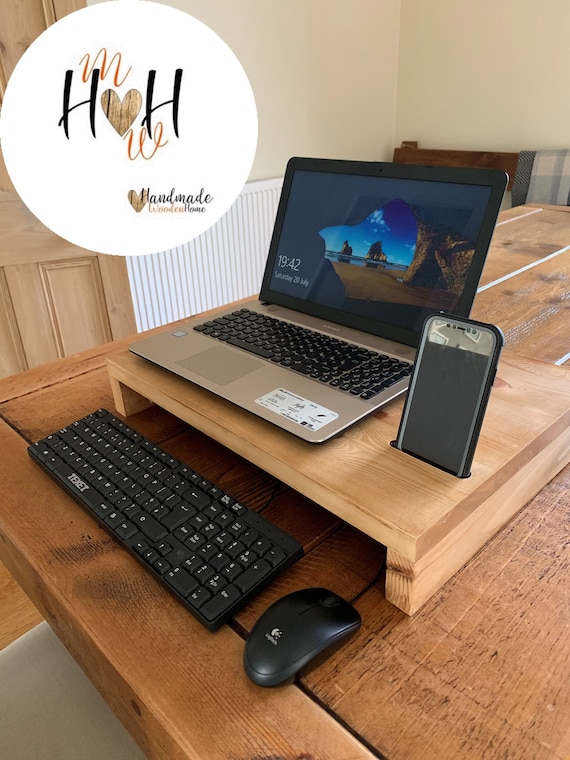The image depicts a neatly organized workdesk setup. At the focal point is a black and gray laptop positioned on a wooden riser that slightly elevates it, providing ergonomic benefits. To the right of the laptop, nestled within a slot on the riser, is a black smartphone. In front of the riser, a black keyboard and mouse are placed for easy access and use. The entire desk is crafted from brown wood, complementing the beige and white walls of the room. A beadboard runs along the lower half of the wall, adding a touch of texture. To the left side of the image stands a brown wooden door.

In the upper left corner of the image, there is an inset with a white circle displaying the text "H heart H" and "M heart W" in red, with the phrase "Handmade" written at the bottom, suggesting an emphasis on artisanal craftsmanship, likely referring to the wooden riser. The stylish setting blends technology and handmade elements harmoniously, illustrating a workspace that is both functional and aesthetically pleasing.